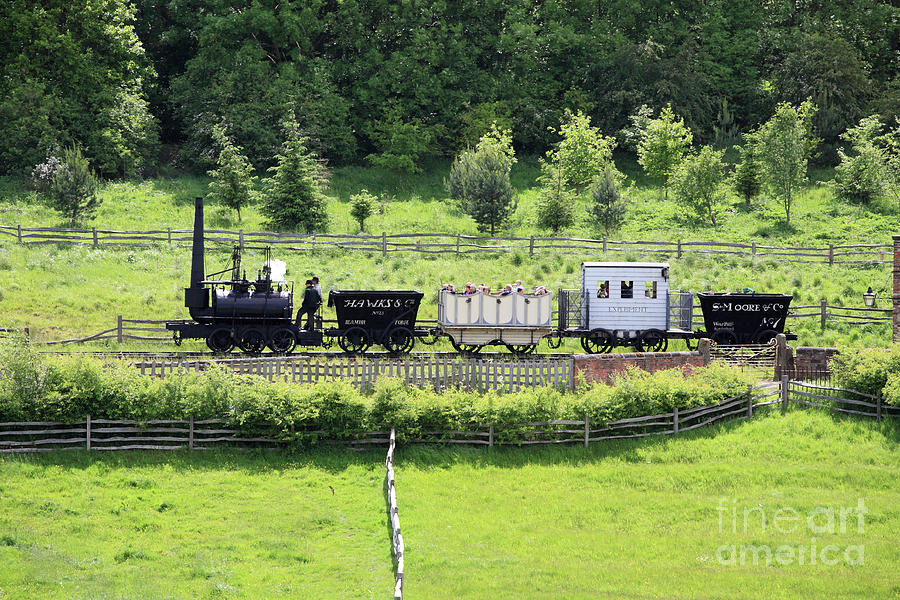In an outdoor landscape mode photograph by Fine Art America, a small, miniature train is depicted, consisting of five varied carriages. The black train engine, about the size of a commercial car or SUV, sits at the front, emitting a puff of white steam, with two individuals standing atop it. Following the engine is a cart marked with "Hawks, Hammer," which leads to a high-walled open-top cart carrying eight to ten passengers with only their heads visible. Behind this is a white-striped cabin-like carriage with a roof, labeled "Smoore, S-M-O-O-R-E, and Co.," appearing like a dumper cart. The entire scene is surrounded by lush green fields, bushes, and trees, with a brown wooden fence running horizontally through the foreground, intersected by an iron gate attached to a red brick wall. The bottom right corner of the image features "Fine Art America," indicating the image's source.